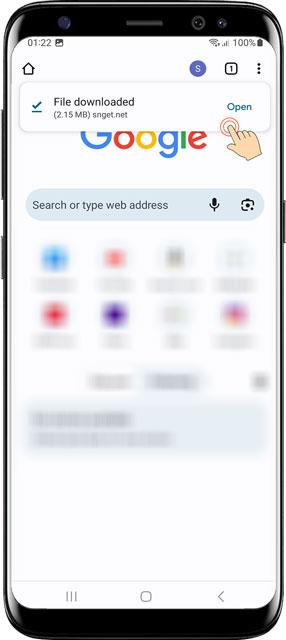A smartphone screen displaying various elements and notifications. The time on the phone is 1:22, and the battery is fully charged at 100%. There is a notification indicating a file has been downloaded, marked with a blue check. The file size is 2.15 MB, sourced from sngnet.net, and there is an option to "open" displayed in blue text. A hand icon pointing with an arrow appears on a rectangular element, along with a house icon, a blue circle with an "S", and a square containing one and three vertical dots. At the top, the Google logo is prominently displayed in its signature colors: a blue "G", a red "O", a yellow "O", a blue "G", a green "L", and a red "E". Below the logo is a search bar with the placeholder text "Search or type web address", accompanied by microphone and camera icons. The main part of the screen shows blurred sections with what appears to be eight apps, and potentially three to four more sections that are also blurred. At the bottom of the screen, there are three navigation icons: three vertical lines, a square, and a left-facing arrow.